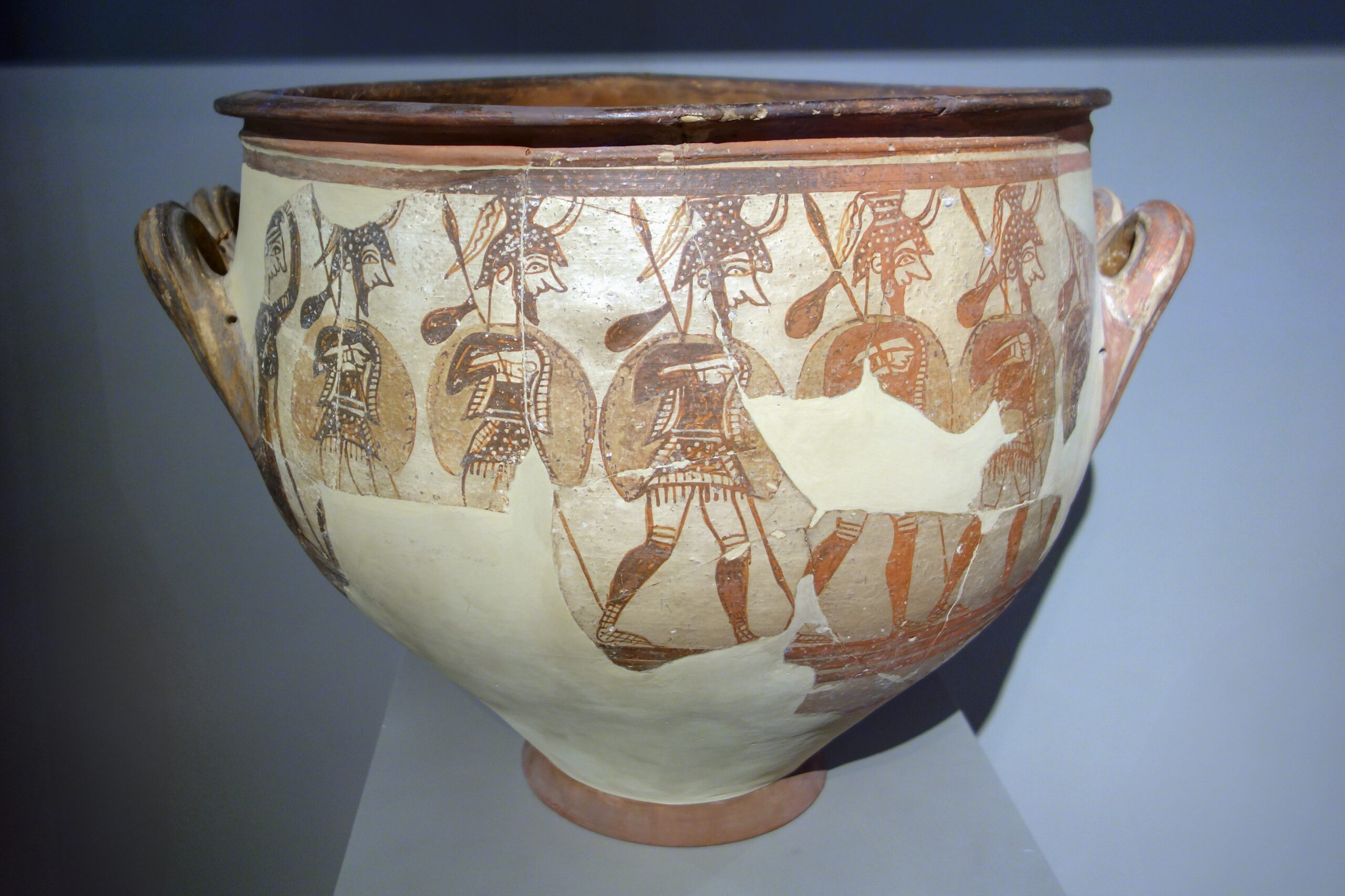The image depicts an ancient, handcrafted ceramic bowl displayed on a shelf, likely in a museum due to its aged and delicate state. The bowl is predominantly tan with a cream-colored glaze and features intricate brown and beige markings. The rim is notably dark brown and slightly uneven, indicative of its handmade origin. The bowl's body broadens significantly from a small base to a wide, flaring lip.

Detailed paintings adorn the sides, showcasing soldiers in various poses. Each soldier is similarly attired, wearing helmets – some with horn-like projections – and skirts, holding spears and shields. Despite the repetitive nature of the figures, slight variations suggest the painter could not replicate them exactly. The bowl also exhibits signs of wear, including cracks and possible repairs, adding to its historical intrigue and value.